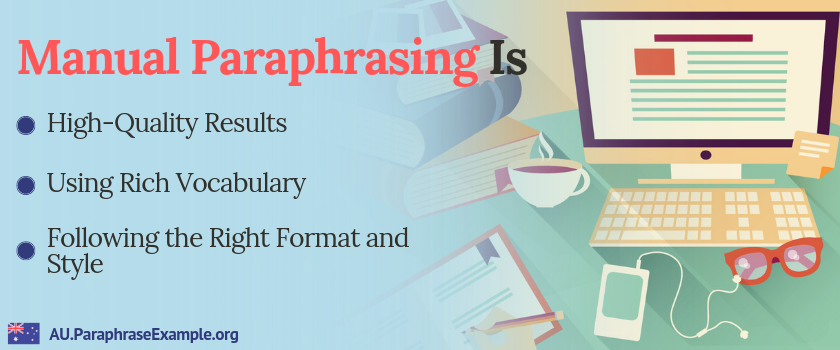The slide features a gradient blue background on the left, transitioning into a digital collage on the right showcasing various items. These items include a clip art of a computer, an old iPod with wired earbuds, a pair of red-rimmed glasses, a steaming cup of coffee, and a small stack of books. On the left side of the slide, the text "Manual Paraphrasing" is prominently displayed in red font, followed by the word "IS" in black font. Underneath, three blue bullet points detail the benefits of manual paraphrasing in black font. The bullet points are: "High Quality Results," "Using Rich Vocabulary," and "Following the Right Format and Style," each word beginning with a capital letter, except for conjunctions and articles. At the bottom left of the slide, "au.paraphraseexample.org" is written in blue font, providing the source of the information.